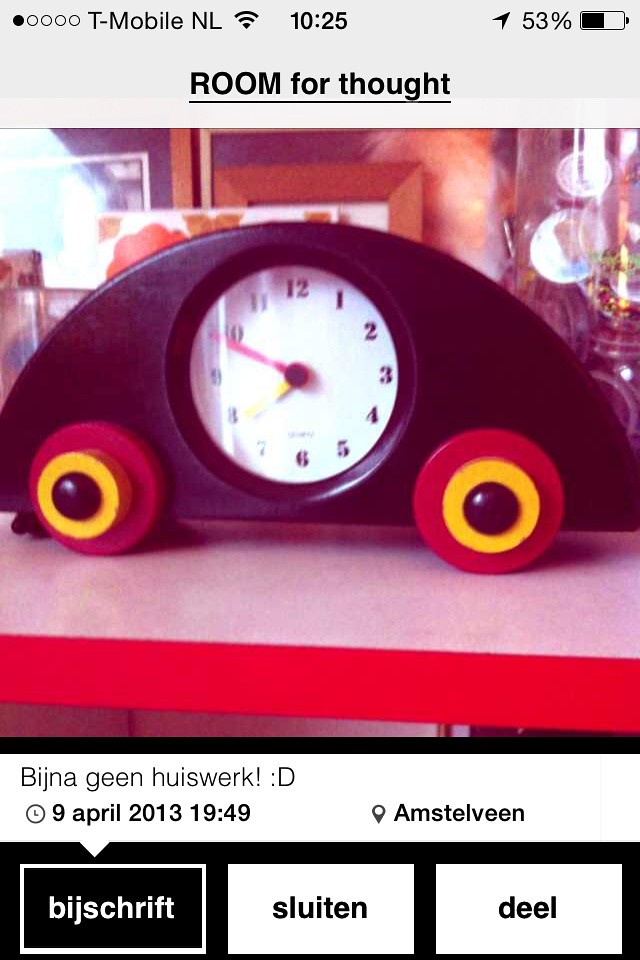The image is a vertical, portrait mode iPhone screenshot showcasing a detailed view of a unique mantel clock. The top of the screen displays the T-Mobile NL network indicator, Wi-Fi signal icon, and the time 10:25 alongside a battery icon showing 53%, which is slightly more than half full. Below this, the screen reads "Room for Thought" in English. The mantel clock, prominently featured, is designed to resemble a toy car with a wooden body, detailed with black, red, and yellow colors. It sits on a gray surface with a red side. The clock's face is positioned where the car's windshield would be, with red and yellow hands showing the time at around 7:50. Black numbers encircle the clock's face. Below the image of the clock, there's text that appears to be in Dutch, mentioning "Benjagijn, who is work" and the date "9th of April 2013," alongside the location "Amstelveen." The bottom of the screenshot features three Dutch words, adding to the overall foreign language theme. Behind the clock, the setting appears to be a bedroom, enhancing the vintage ambiance of the image.